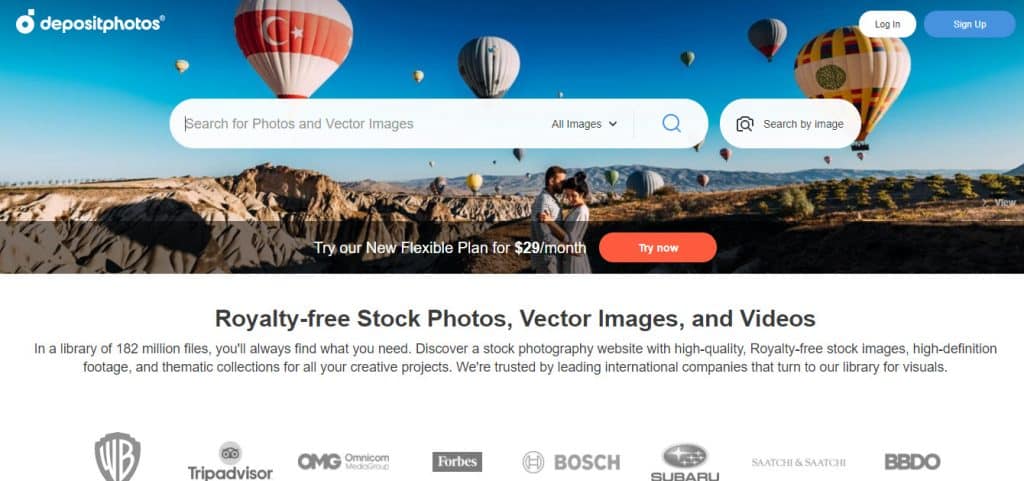This is a screenshot of the home page of the DepositPhotos website. The background features a visually captivating scene with several uniquely designed hot air balloons. The top section of the page includes navigation options: "Log In" and "Sign Up." Below these, a prominent search bar invites users to "Search for photos and vector images," offering options to "Search by image" as well. There's a highlighted promotional banner encouraging visitors to "Try our new flexible plan for $29 a month - Try Now."

The website promises a vast library of 182 million files that includes "royalty-free stock photos, vector images, and videos," ensuring you'll "always find what you need." Descriptive text promotes the platform's high-quality stock images, high-definition footage, and thematic collections, ideal for various creative projects. It highlights that DepositPhotos is trusted by leading international companies for visual resources.

At the bottom of the page are logos of various notable clients, including Warner Brothers, TripAdvisor, QMG, Forbes, Bosch, Subaru, BBDO, and Snatch and Sketch.